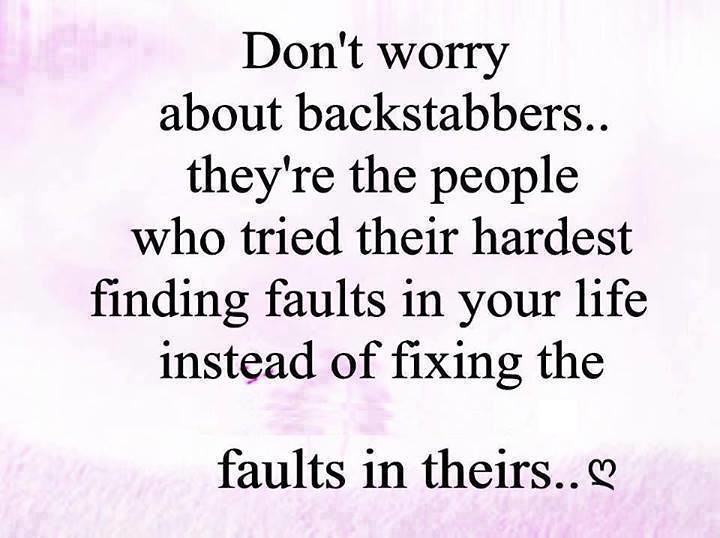The image is a meme or inspirational quote with a predominantly pink and purple gradient background. The text, written in a mix of upper and lower case black font, is centered both horizontally and vertically. The quote reads: "Don't worry about backstabbers... They are the people who tried their hardest finding faults in your life instead of fixing the faults in theirs..." A violet heart symbol follows the text, adding a decorative touch. The overall design and structure are minimalist and clean, with the message emphasized through its straightforward presentation and the heart symbol at the end.